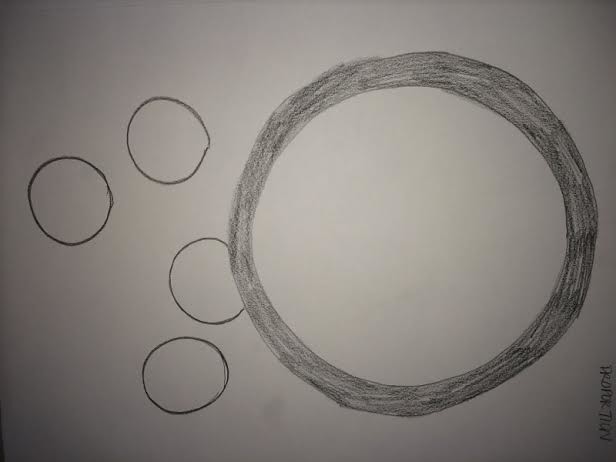**Detailed Caption:**

A hand-drawn sketch on a blank, white sheet of paper devoid of any lines or markings. On the left side, there are four distinct, imperfect circles, each slightly larger than a silver dollar, drawn with what appears to be a pencil. The circles are arranged as follows: 

- The first circle is positioned on the far left.
- The second circle sits about half an inch to the right and slightly above the first one.
- The third and fourth circles are located towards the bottom, aligned almost vertically with only about a half centimeter gap between them. 

The third circle is also connected to a significantly larger circle, approximately five times the size of the smaller ones. The edge of this large circle is shaded in pencil, creating a stark contrast with its untouched, white interior. The entire drawing maintains a monochromatic theme, relying solely on pencil shading for depth and definition.